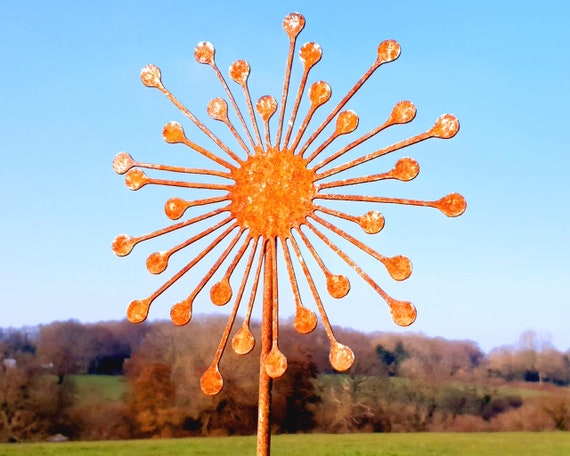This image features a detailed close-up of a decorative garden ornament designed to resemble a sunburst or flower, staked into the ground in a wide, flat grassland. The metallic ornament, once possibly silver, now sports an orange hue due to rust from exposure to the elements. The ornament has a central sun or flower design, with long rays extending outward, each ending in larger, rounded nodes. The photograph, taken during the day, captures a bright blue, cloudless sky above a backdrop of autumn-colored trees and small hills. The foreground showcases lush green grass, with the vibrant, rusted ornament standing out prominently. The scene is devoid of people or animals, focusing purely on the aged yet charming lawn ornament and its serene natural surroundings.